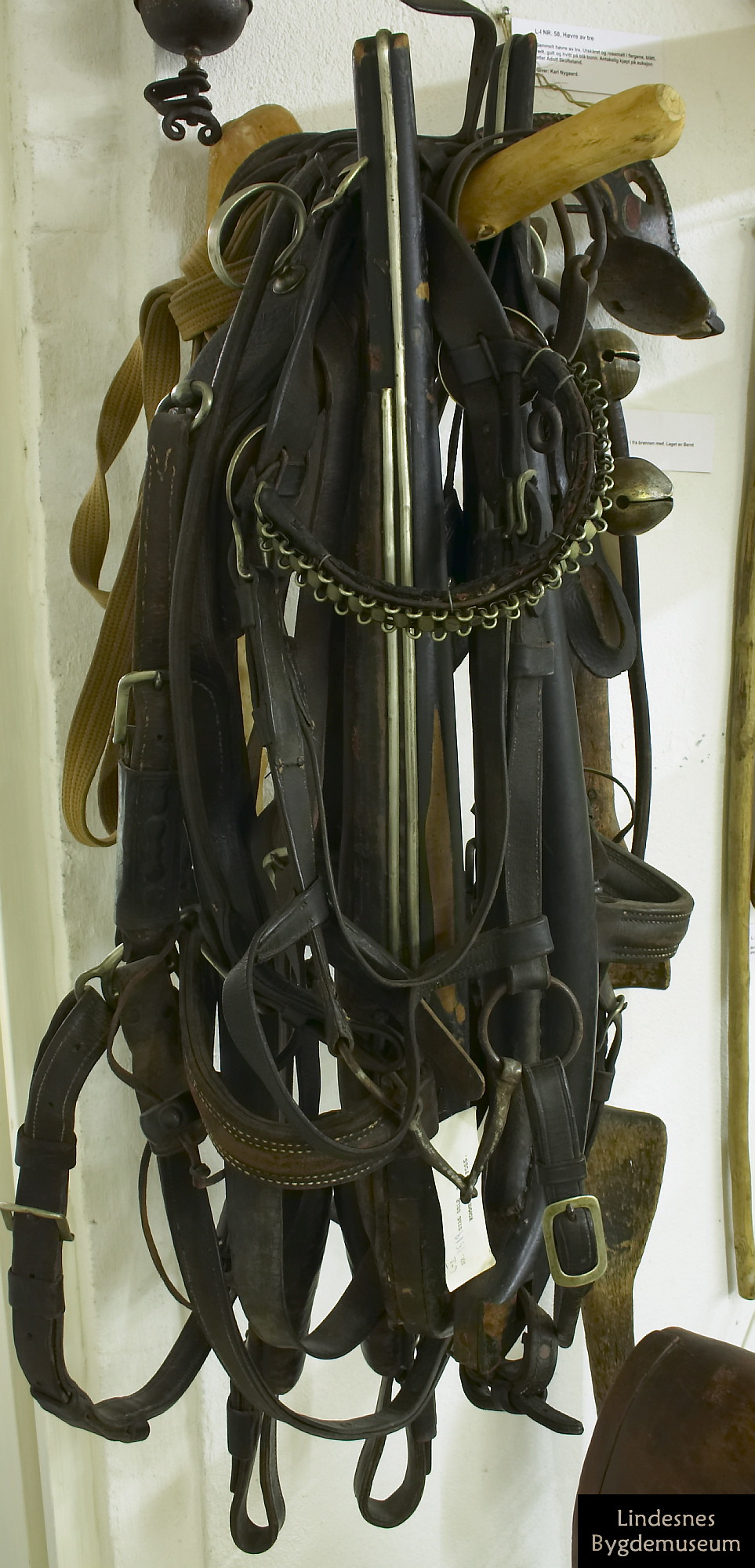The photograph captures a bright, indoor setting with an abundance of natural light streaming in, likely from a nearby window. Dominated by a clean, white wall, the scene focuses on a hook jutting out, clearly handcrafted from a knotted piece of wood, finished with a light honey-colored stain. This rustic hook serves as a support for an array of equestrian gear, including bridles, halters, and harnesses, most of which are made of leather in various shades of black, tan, and dark brown. Some of these pieces feature metal studs, adding a touch of detail to their utilitarian design. Among the tangled assortment hangs a set of bells, commonly used in horse equipment. In the bottom right corner of the image, there is a dark brown object partially visible and a small, unreadable print on a black block. Additionally, barely discernible to the far right, a brown stick-like object is suspended on the wall, adjacent to a white label with black text that is too small to read.